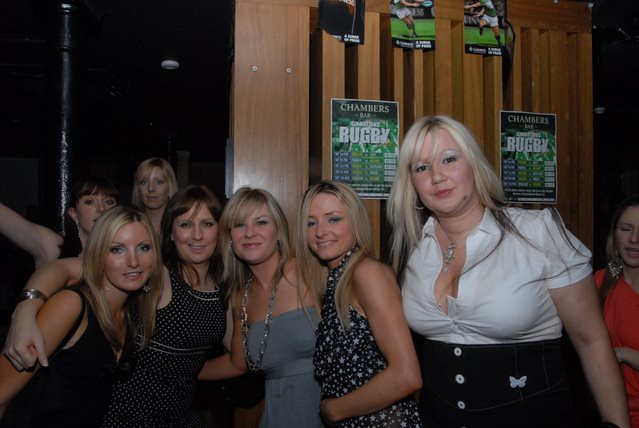This is an indoor photographic image featuring a group of seven white women posing closely together. They are dressed in various stylish outfits, primarily in dresses, and are positioned against a wall adorned with posters that include images of soccer players. Central to the backdrop is a sign reading "Chambers Rugby" along with some unreadable text regarding dates.

From right to left, the women are as follows:

1. A young white woman in a red dress, slightly out of the main group, indicating she might not be part of the posed photo.
2. A blonde woman wearing a white shirt and a black skirt with white buttons, complete with a butterfly design.
3. A thin blonde woman in a black sleeveless dress decorated with white stars.
4. Another thin blonde woman in a sleeveless gray dress, accessorized with a long necklace.
5. A brunette woman with brown hair, sporting a black and white polka-dot dress, and wearing a bracelet.
6. A thin blonde woman in a black sleeveless dress, being held by the woman in the polka-dot dress.
7. In the background, there is a woman with dark hair wearing a sleeveless dress, although the dress's details are obscured.
8. Also in the background, slightly above the dark-haired woman, is the head and shoulders of a blonde woman whose clothing is not visible.

The women appear united and close-knit, with some of them leaning on each other or having their arms around each other's shoulders. The overall atmosphere suggests a celebratory gathering, possibly at a bar, given the reference to rugby flyers and the "Chambers Rugby" sign on the wall.